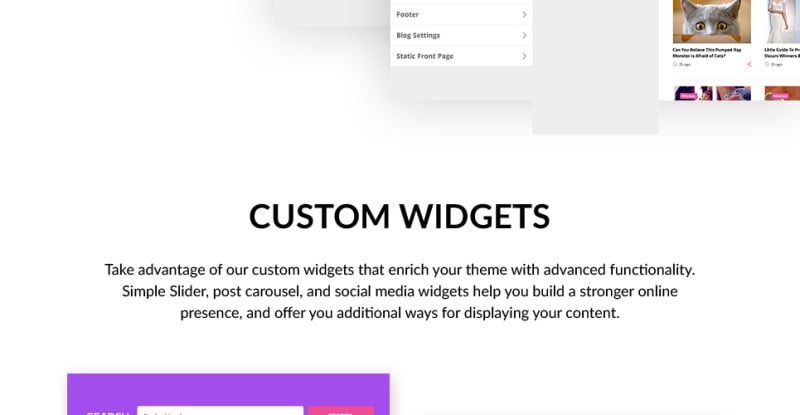This image is a screenshot of a webpage titled "Custom Widgets." The title, "CUSTOM WIDGETS," is prominently displayed in bold, uppercase black text at the center of the page. The webpage features a primarily white background with black text, offering an elegant and clean look. Directly below the title, a description reads, "Take advantage of our custom widgets that enrich your theme with advanced functionality. Simple slider post carousel and social media widgets help you build a stronger online presence and offer you additional ways for displaying your content." 

The bottom left corner of the screenshot shows a section that has been redacted and obscured within a purple, opaque rectangle, indicating concealed content. Additionally, at the top center of the image, a small window appears with options labeled "footer," "blog settings," and "static front page," highlighting navigation or customization settings for the webpage. This window features a white background with gray shading, providing a subtle contrast to the page's overall design.